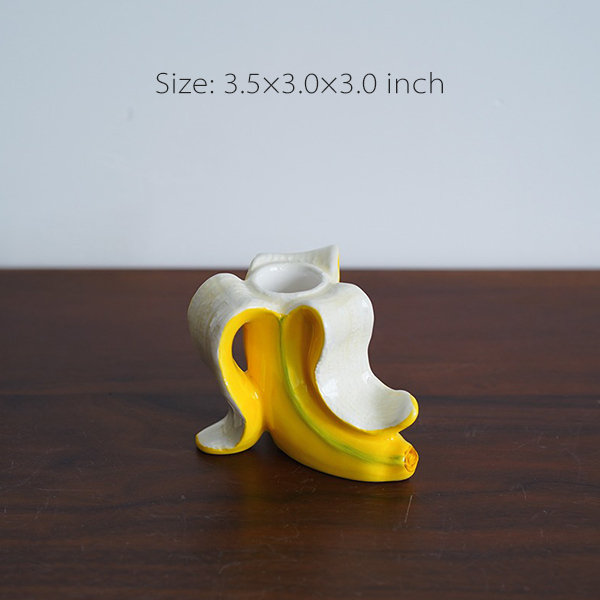A detailed close-up image shows a ceramic banana holder with dimensions of 3.5 x 3.0 x 3.0 inches, as indicated by black font text at the top of the picture. The holder, resembling a half-peeled banana, is upright with a slightly curved base. The banana peel is yellow with subtle green veins, while the inside is white. The center of the banana is hollow, suggesting it can be used as a candle or pen holder. This whimsical piece is positioned on a dark brown wooden desk, showcasing distinctive black wood swirls. The background is a light gray, possibly from a wall or wallpaper.